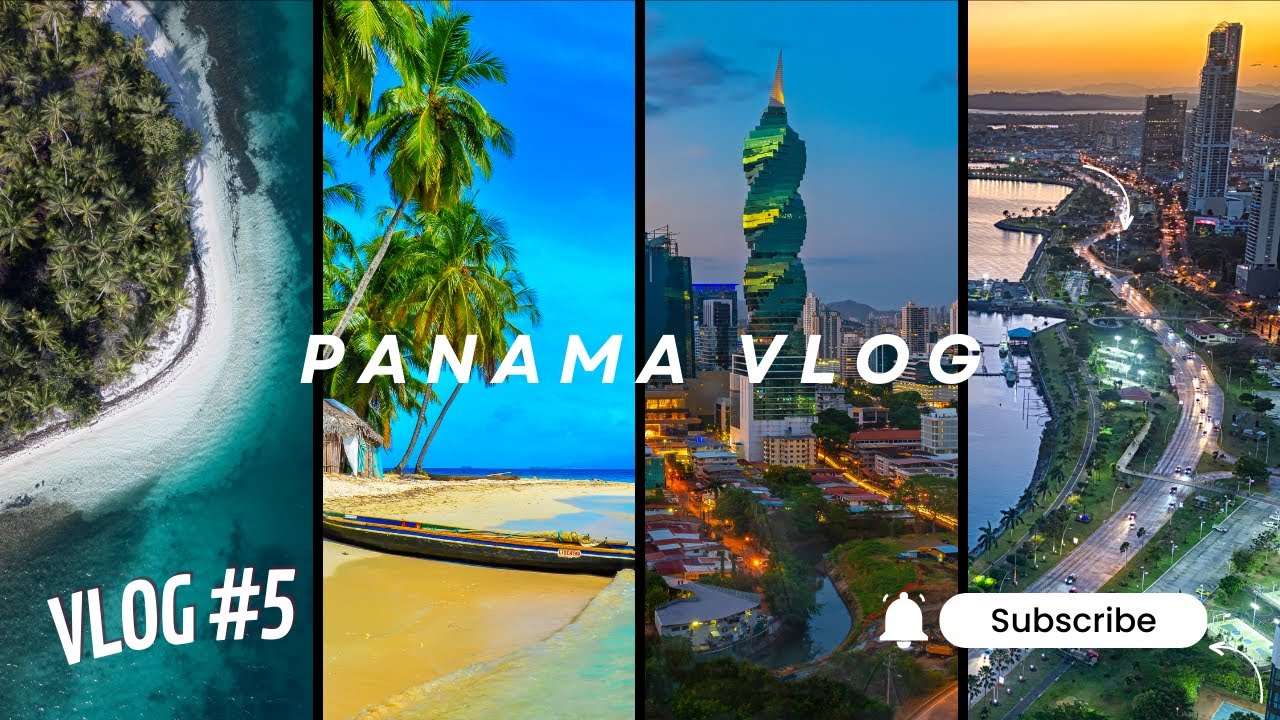The image depicts a screenshot of a blog page dedicated to travel destinations, with a particular focus on Panama. The central feature of the page is bold white text that prominently reads "Panama Blog," indicating the geographical focus of the content. The background includes a diverse array of visuals representative of various locations in and around Panama.

On the lower right-hand corner, adjacent to an urban cityscape, is an oval-shaped button with black text that reads "Subscribe." Beside this button is a notification bell icon with two hash marks, suggesting an alert or ringing function, possibly hinting at a YouTube or similar social media platform where users subscribe for updates.

The cityscape depicted is bustling with many roads filled with traffic, surrounded by large buildings in shades of gray, dark brown, and black, illuminated by numerous city lights. 

To the left, a picturesque image of a small island showcases tall, dark green palm trees surrounded by white sandy beaches and water in beautiful shades of dark blue, cyan, and teal. This visual vignette exudes a tropical feel, emphasizing natural beauty and tranquility.

At the lower left, bold white text announces "Blog #5 VLOG," accompanying a close-up of another idyllic beach scene. This scene features palm trees varying from dark green to light green with hints of yellow, under a bright, sunny sky with dark and cyan blue hues mixed in. The beach's golden-brown sand transitions to white as it nears both the hut on the left and the shimmering ocean waters. 

A distinct architectural detail within the scene includes a tall, spire-like structure resembling an ice cream cone, painted in teal with yellow accents and capped with golden brown. This building stands amidst a cityscape composed of skyscrapers in shades of gray, black, brown, and tan, interspersed with vibrant city lights and dark green trees.

Through its rich imagery and descriptive elements, the page vividly encapsulates the allure and diversity of Panama as a travel destination.